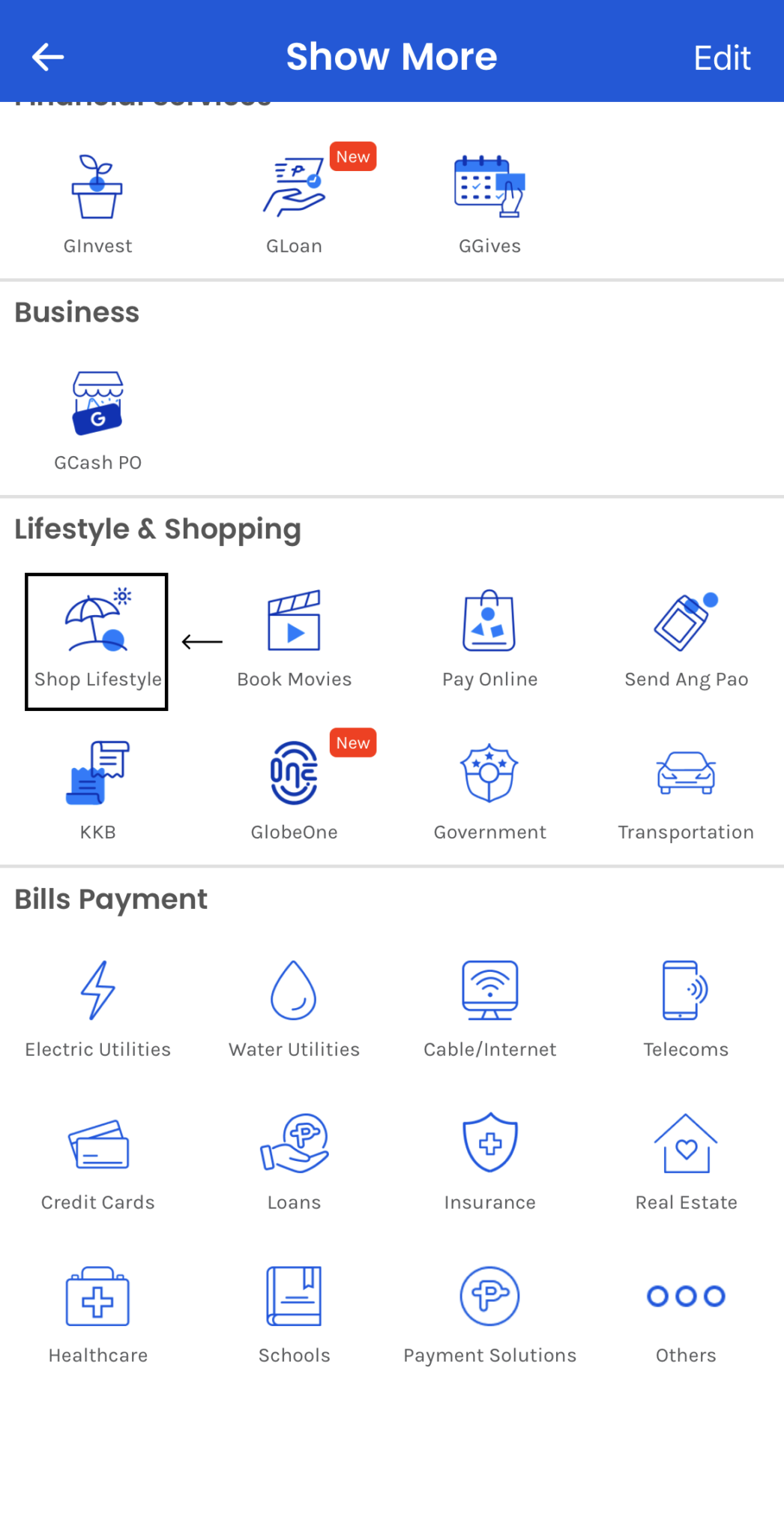This image is a detailed screenshot taken in portrait mode, likely from a phone. The interface has a blue top stripe which includes three elements: a back arrow in the upper left corner, a bold "Show More" text in the center, and an "Edit" option in the upper right corner.

Below the top stripe, the background is white and is organized into multiple categorized rows. 

The first row contains three items: "GinVest," "G-Loan" (highlighted with a red rectangle), and "G-Gives." 

A horizontal line separates this row from the next, which lists: "Business," "G-Cash," and "P.O."

Another horizontal line follows, leading into the "Lifestyle and Shopping" section. This section features two rows of four columns each, with categories as follows:
- Row 1: "Shop Lifestyle" (currently selected, indicated by a bolded square with an arrow pointing to the selection), "Book Movies," "Pay Online," and "Send Ang Pao."
- Row 2: "KKB," "Globe One" (highlighted with a new rectangle), "Government," and "Transportation."

Below this section, there is another category titled "Bills Payment," featuring three rows of four columns:
- Row 1: "Electric Utilities," "Water Utilities," "Cable," and "Internet," "Telecoms."
- Row 2: "Credit Cards," "Loans," "Insurance," and "Real Estate."
- Row 3: "Health Care," "Schools," "Payment Solutions," and "Others."

The screenshot appears to show a well-organized interface, likely displaying various user service options on a mobile application or website.